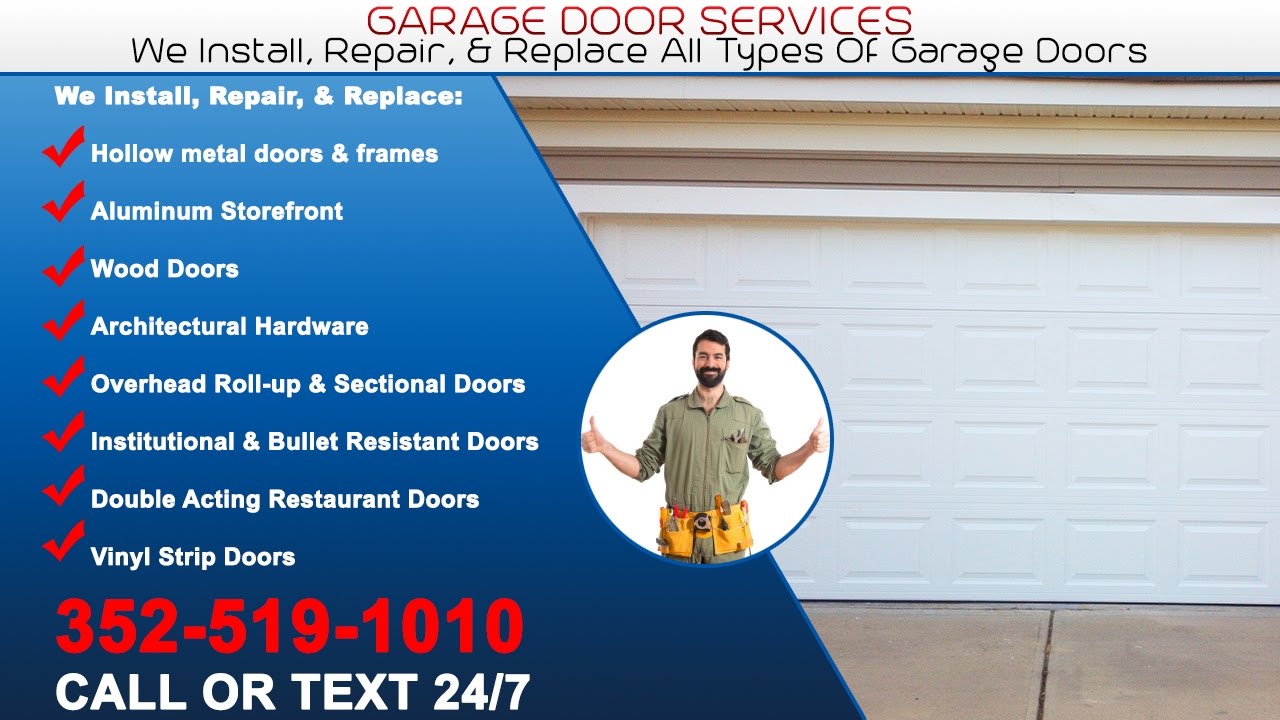The image depicts a promotional advertisement for a garage door service company. Dominating the image is a large, two-car garage door adorned with rectangular panels from top to bottom and side to side, set against a house exterior featuring tan and brown accents. A smooth concrete driveway leads up to the garage.

Center-stage, a red banner prominently displays the service offerings: "We Install, Repair, and Replace All Types of Garage Doors." This text is accentuated by contrasting black and white fonts for emphasis.

On the left side, a section shaded in blue diagonally crosses the lower part of the garage door and features a smiling man equipped with a tool belt, giving a thumbs-up. He sports a beard, mustache, and a green shirt, projecting a friendly and professional image.

Inside the blue section, a checklist details the comprehensive services provided:
- Hollow metal doors and frames
- Aluminum storefronts
- Wood doors
- Architectural hardware
- Overhead roll-up and sectional doors
- Institutional and bullet-resistant doors
- Double-acting restaurant doors
- Vinyl strip doors

Alongside the detailed list, a bold, red phone number coupled with "Call or Text 24-7" written in white assures potential customers of round-the-clock availability.